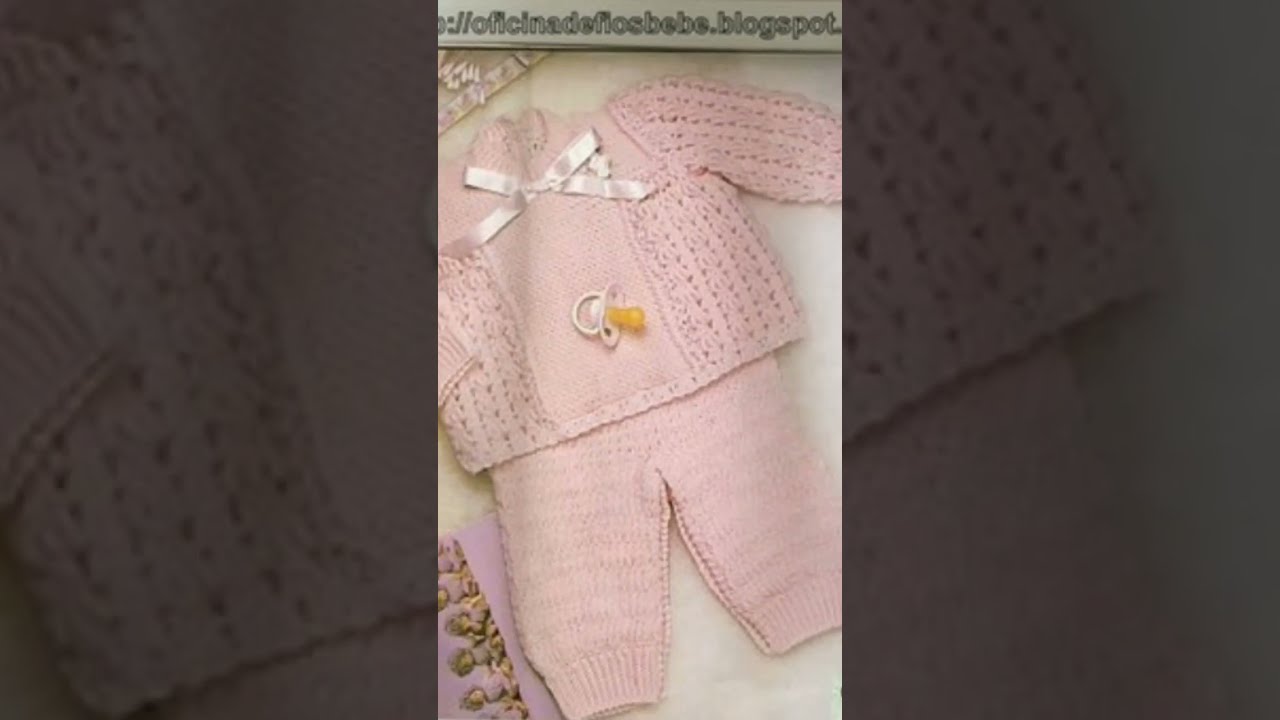The image features a meticulously handmade, knitted baby girl's outfit in a delicate pale pink hue. The ensemble includes a long-sleeved top adorned with a white, velvety ribbon at the neckline, adding a touch of elegance. The knit texture of the top is slightly more intricate around the sides and shoulders, creating a visually appealing detail. It is paired with matching knitted pants that taper at the cuffs. A white bib with a yellow pacifier clipped onto it rests on the shirt, enhancing the outfit's charm and practicality. The entire set is carefully laid out on a beige surface, alongside a greeting card in the lower left corner. The image background is cropped with black and white borders, suggesting that it was captured from a video. A website URL, "oficinadeflosbebe.blogspot.com," is displayed at the top, indicating where similar custom-made outfits can be purchased for an upcoming baby or grandchild.